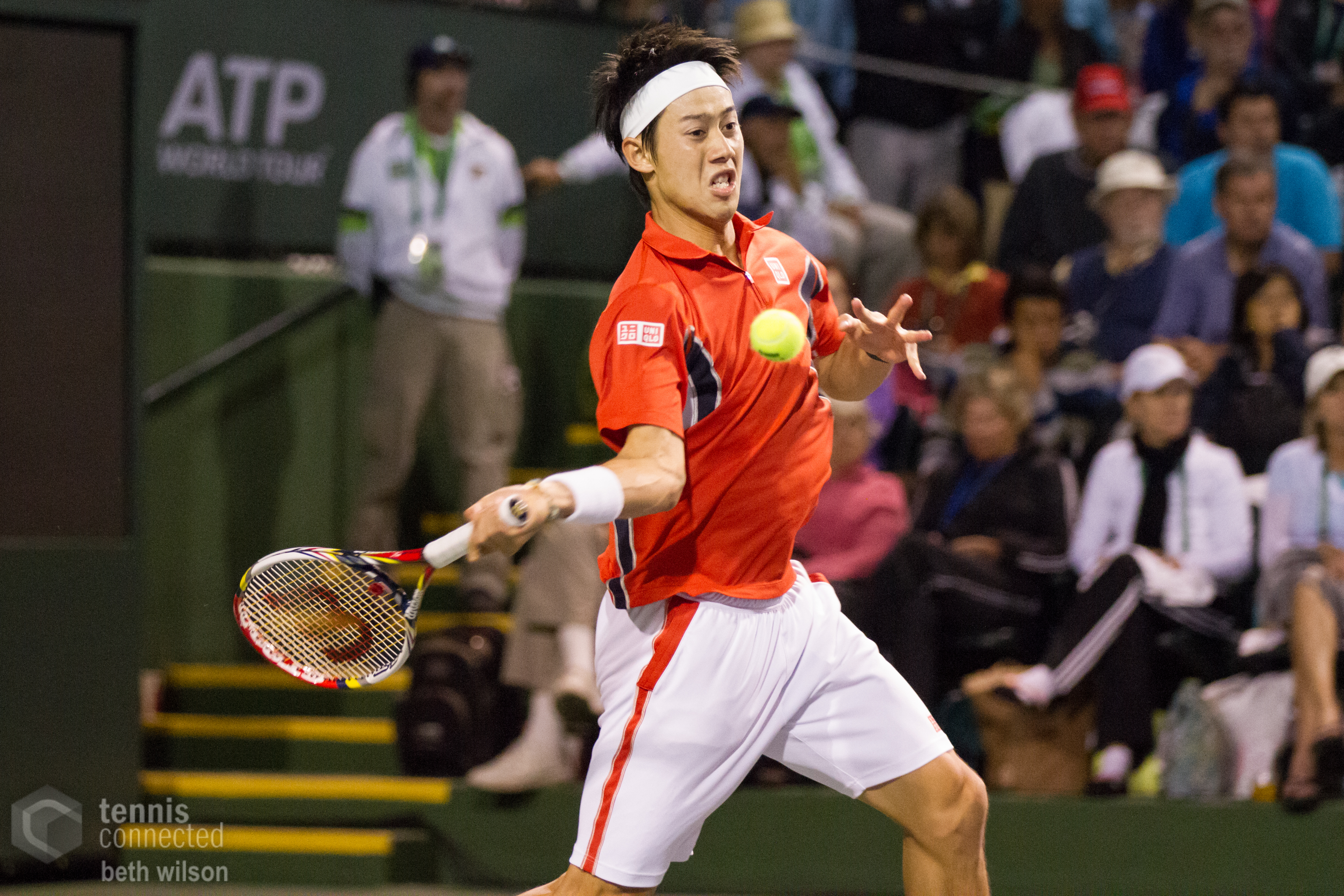In the image, a tennis player is captured in action at an outdoor tennis court during the daytime. Positioned centrally, the athlete is clad in a complete tennis outfit and holds a tennis racket in his right hand, ready for his next move. The crowd in the background is seated on elevated bleachers, accessible by a visible staircase leading up to their seats. A variety of colors, including black, green, gray, red, orange, light blue, light green, and pink, are prevalent throughout the scene, adding vibrancy. The bottom left corner of the image features a watermark that reads "Tennis Connected, Beth Wilson."